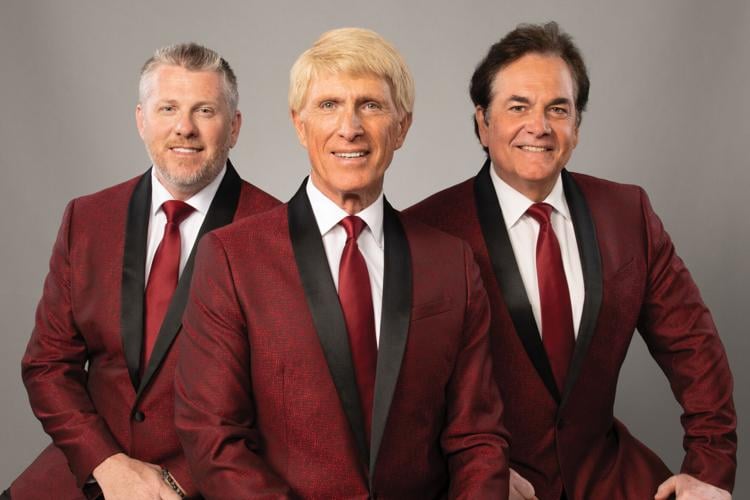In this photograph, three men are seated closely together, smiling directly at the camera. They are all dressed uniformly in dark red suits with black outlines, white shirts, and red ties. Each man has his own distinct hair color: the man on the left has short grey and brown hair with a short beard and mustache, the man in the middle has light brown hair, and the man on the right has dark brown hair. The background is a simple, empty mix of white and light grey. Their upper bodies are clearly visible, but their lower bodies and the seats they are on are not shown. The coordinated attire and their joyful expressions suggest that they might be performers or professionals posing for a formal group shot.